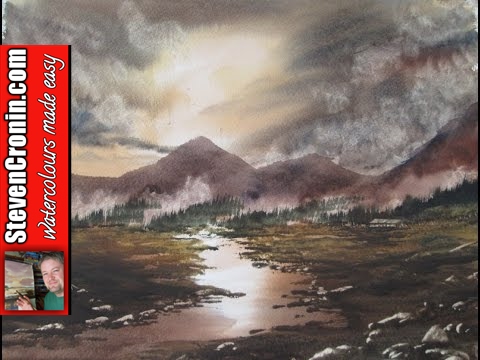The image is a detailed watercolor painting depicting a serene mountain valley scene. Dominating the background are dark, brown-hued mountains that form a rugged range, with mist shrouding the forested area at the base. In the foreground, a calm body of water, possibly a river or lake, meanders through a verdant expanse of green grass. The water reflects the soft light of the sun, which is breaking through a cloudy, overcast sky colored in grayish-brown tones, adding a subtle glow to the otherwise muted color palette of beiges, browns, and forest greens. 

On the far left of the image is a prominent red label with white text that reads "stevencronin.com" and "Watercolors Made Easy," accompanied by a picture of a man, presumably Steven Cronin himself, standing beside what appears to be the very painting showcased here. The overall atmosphere of the painting is somewhat gloomy, yet the sun's light on the water brings a touch of brightness to the scene. The presence of the label and the image of Steven Cronin indicates that this painting is likely part of an advertisement for an instructional watercolor painting video or tutorial series.